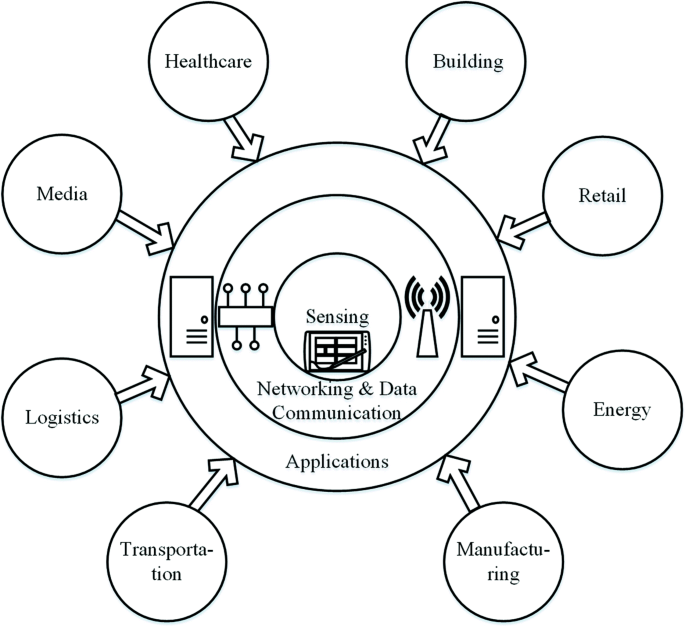This image features a detailed organizational diagram of a business. At the center, there are three nested circles. The innermost circle is labeled "sensing" and depicts what looks like electronic equipment with joysticks and a Wi-Fi signal symbol. This central area is surrounded by a middle circle labeled "networking and data communication." Outside of this is the outer circle labeled "applications," which includes icons resembling paperwork on either side.

Encircling the outermost ring are eight smaller circles, each connected to the central configuration with arrows. These smaller circles are evenly spaced, each containing a word representative of different sectors: starting from the top and moving clockwise, they read "building," "retail," "energy," "manufacturing," "transportation," "logistics," "media," and "health care." This arrangement visually represents how various sectors integrate into the core functions of sensing, networking and data communication, and applications.